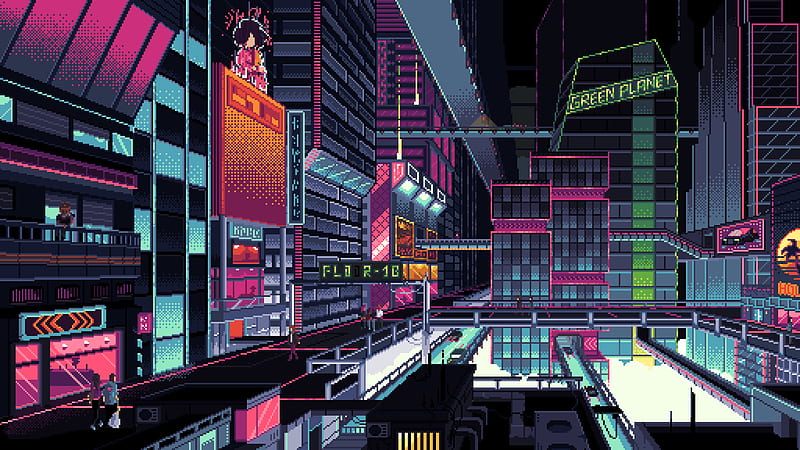The image portrays a meticulously detailed, pixelated art representation of a futuristic, cyberpunk-inspired cityscape, reminiscent of a dystopian Tokyo. The scene is filled with towering gray buildings adorned with vibrant digital advertisements, including a prominently displayed sign that reads "Green Planet." The city is bathed in hues of pink, purple, and green, adding to its retro-futuristic aesthetic. Multiple levels are visible in the city: elevated walkways populated by pedestrians, and below that, streets bustling with vehicular traffic. A monorail track or subway can also be seen below the street level. The overall impression is of a complex, neon-lit urban environment featuring elements like high-tech billboards, including one showcasing a race sports car, and various people moving through this animated, electronic world.